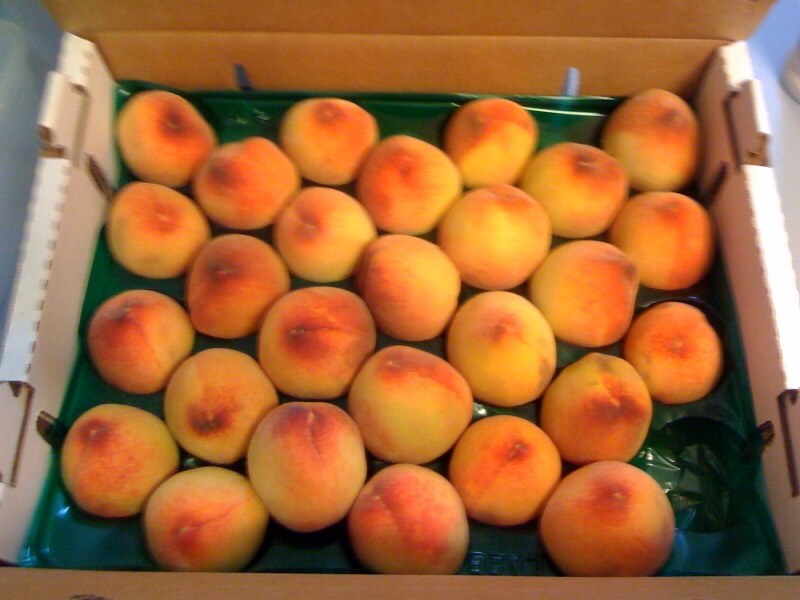The image is a slightly blurry photograph featuring an open white cardboard box containing 27 peaches. The box, which reveals a light brown on the inside of the lid, houses the peaches in a light green, cushioned plastic tray. Each peach, exhibiting unique characteristics, varies in a yellowish-orange hue with darker spots and some bruising, complemented by red and pink patches around the center. The tray's layout is organized into rows of four, and a single space in the bottom right corner is conspicuously empty, suggesting one peach has been removed. The image is taken from a top-down perspective, filling the frame with the details of the colorful, ripe peaches against their green holder.